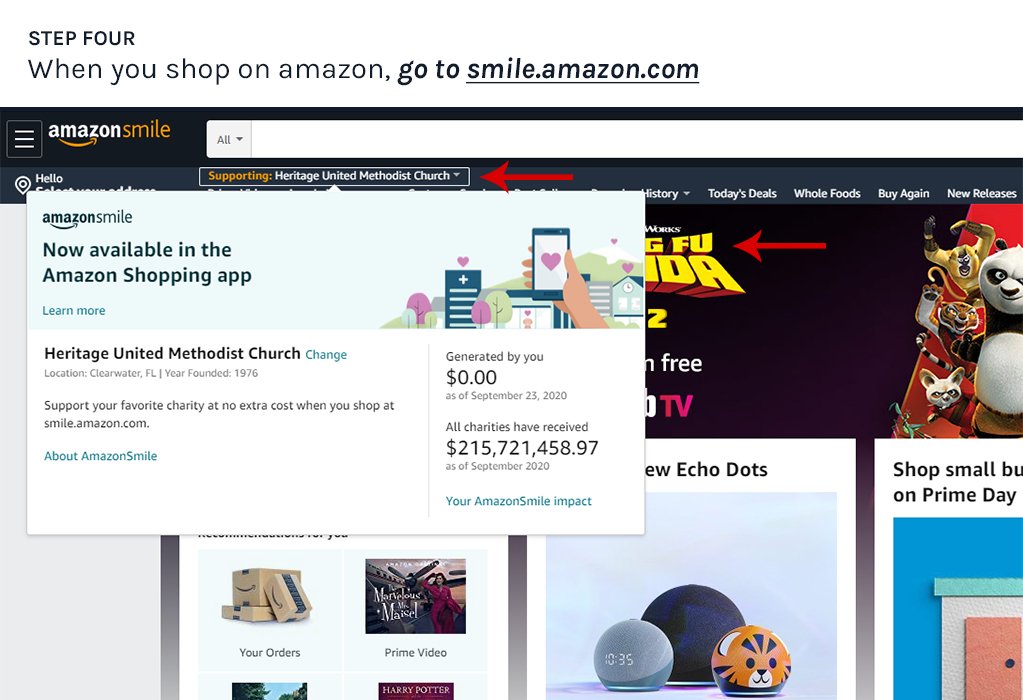Screenshot of the Amazon Smile website during Step 4 of the setup process. At the top, it instructs users to shop via "smile.amazon.com," with the URL underlined. The top left corner features the "Amazon Smile" logo, adjacent to three clickable horizontal bars. Below the logo, it greets the user with "Hello," though the rest of the message is obscured. An arrow points to "supporting Heritage United Methodist Church." A pop-up details that "Amazon Smile is now available in the Amazon shopping app." It emphasizes supporting your favorite charity at no extra cost when shopping on smile.amazon.com. To the right, it shows, "Generated by you: $0 as of September 23rd, 2020," while below, it states that "All charities have received $215,721,458.97 as of September 2020." In the background, there is an ad for "Kung Fu Panda 2" and visible links for "View Echo Dots," "Your Orders," and "Prime Video."